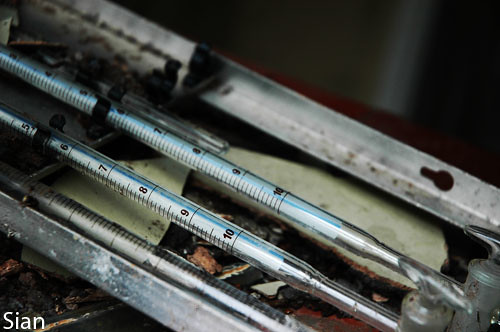The image depicts a set of three tire pressure gauges, though initially there's some ambiguity with syringes. On the bottom left corner, the word "S-I-A-N" is marked with a signature beneath it. There are distinct darker lines near the top end of the gauges. Silver bars are located on both the left and right sides of the image. The central two gauges have visible markings from 5 to 10, with each unit further divided by nine smaller interval lines. The interior of these gauges is primarily white with subtle blue accents, containing a movable black indicator that displays the pressure. A partially obscured third gauge is situated to the left of the central pair. The background features rusted metal with weathered, gaping keyhole-shaped openings and signs of heavy corrosion, especially noticeable on the right and upper parts of the image. The metal ends of the tire pressure gauges also exhibit significant rust, indicating they have been subjected to extensive wear and aging.